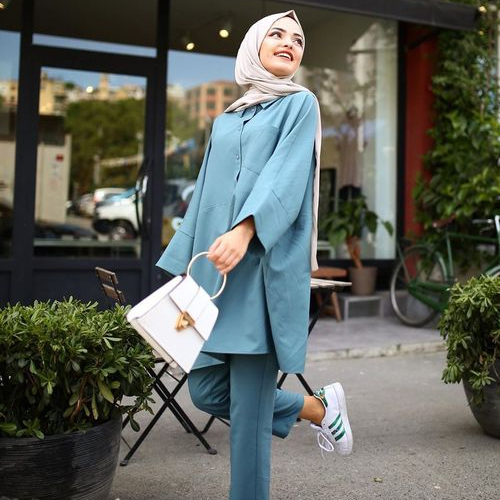The image captures an outdoor scene featuring a woman of possible Arab descent. She is elegantly dressed in a sky blue pantsuit paired with a matching hijab, and she exudes a joyful demeanor with a bright smile on her face. Her right foot is lifted behind her at an angle, showcasing her white Adidas sneakers adorned with green stripes. In her left hand, she holds a chic white handbag accented with a gold clasp. She gazes upwards towards the sky, adding a sense of wonder and delight to the scene. The background includes an array of shrubs, planters, and a few trees, suggesting she is near the front of a building with large glass windows. Reflections in the glass hint at high buildings and cars in the vicinity. Additionally, there is a black bike and a couple of chairs visible, contributing to the lively yet serene atmosphere. The bright natural daylight enhances the clarity and warmth of the image.